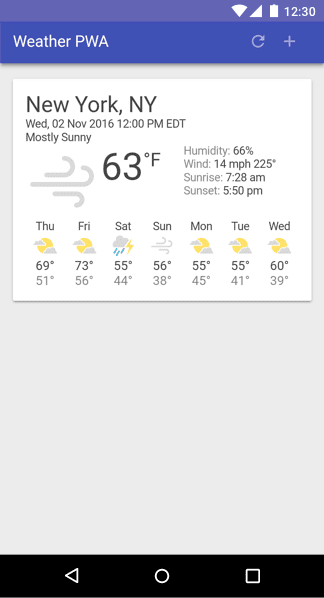This image is a screenshot taken from a smartphone. At the very top of the image, the status bar has a purple gradient background and indicates a full Wi-Fi signal, full phone signal, and a full battery icon. The time displayed on the phone is 12:30. 

Beneath the status bar, there is a weather widget (PWA) highlighted in a blue rectangle with circular arrow and plus sign icons. 

Below this, a white box provides detailed weather information for New York on Wednesday, November 2nd, 2016 at 12 PM EDT. The temperature is displayed as 63 degrees Fahrenheit, with a humidity of 66%, and wind speed of 14 miles per hour coming from 225 degrees. Sunrise is listed at 7:28 AM, and sunset at 5:50 PM.

The widget also features a weekly weather forecast, beginning from Thursday and ending on Wednesday. The forecast starts with a high of 69 degrees on Thursday and shows a low of 60 degrees for the following Wednesday.